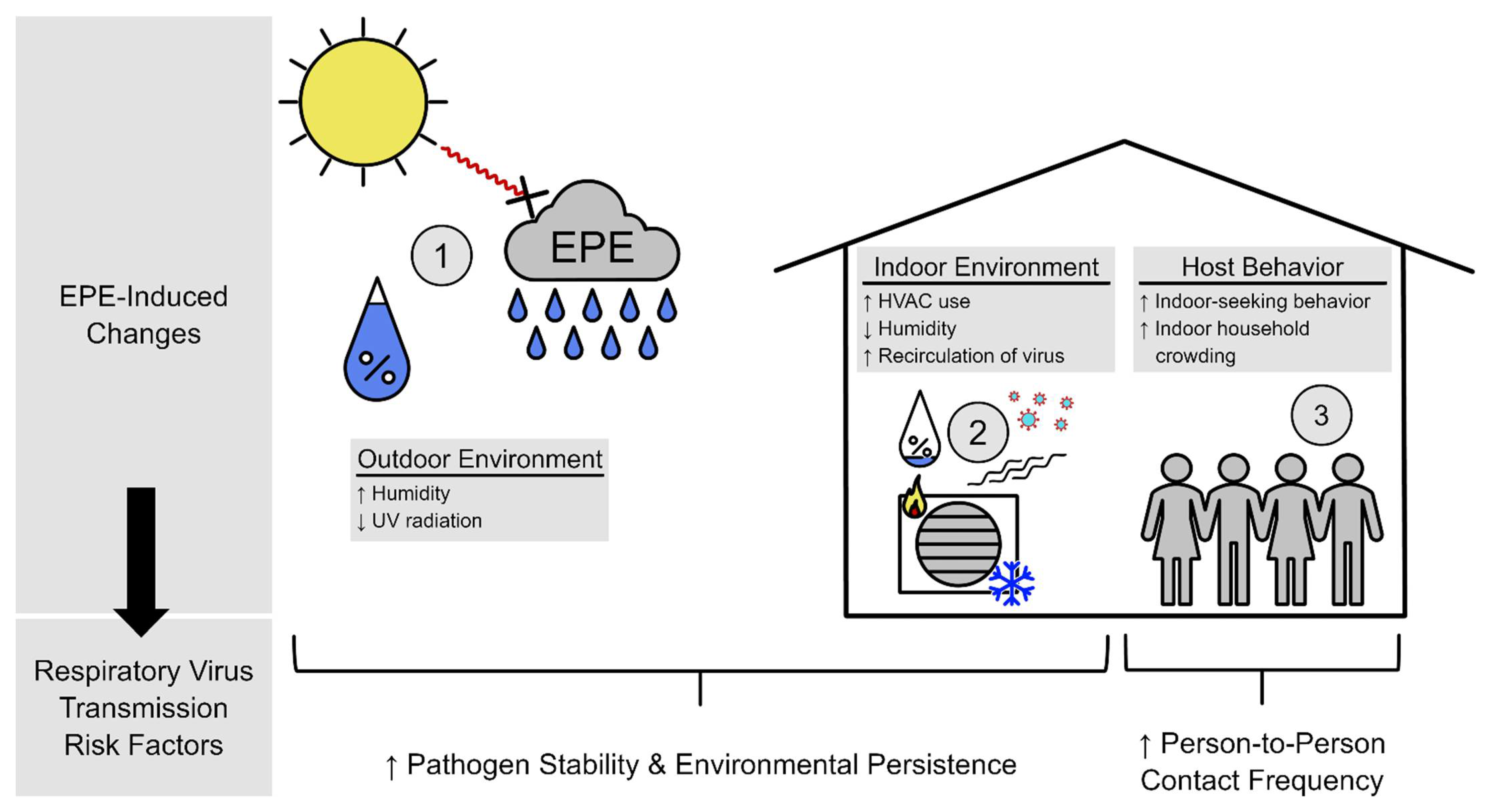The image is a detailed diagram illustrating EPE-induced changes and respiratory virus transmission risk factors. On the left side, a gray rectangle labeled "EPE-induced changes" points down to another labeled "respiratory virus transmission risk factors." A yellow sun in the upper left corner emits red squiggly lines toward a dark cloud marked "EPE," from which blue droplets fall. Below this, the words "outdoor environment" are underlined, with arrows indicating increased humidity and decreased UV radiation. A large blue droplet next to a gray circle with the number "1" signifies these changes.

To the right, a sketch of a building's interior represents the "indoor environment," highlighting increased HVAC use, decreased humidity, and increased recirculation of the virus. Labels point out "host behavior," with arrows indicating increased indoor seeking behavior and indoor household crowding. Profiles of drawn humans next to a gray circle with the number "2" emphasize the crowded indoor settings. In the lower right corner, the diagram illustrates "pathogen stability and environmental persistence," alongside "person-to-person contact frequency," underlined and pointing to the interior structure with a number "3" nearby. The overall poster is on a white background, presenting a complex view of how environmental and behavioral factors influence viral transmission.